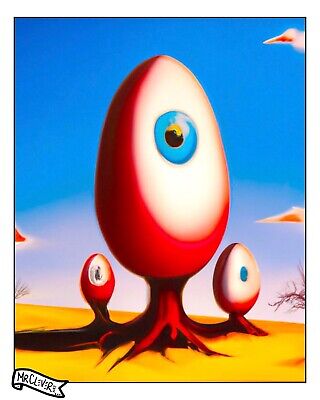This surreal painting features three peculiar tree-like structures emerging from a flat, yellow desert landscape. Each tree has a large, egg-shaped red pod instead of foliage, with each pod housing a single, detailed eyeball. The central pod is notably larger than the others, housing an eye with a white outer area, a blue iris, and a black pupil. The flanking pods on either side are smaller but share these color characteristics. The sky above is mostly clear, with some hazy cloud formations near the horizon and three distinct red clouds—two on the right and one on the left. To the right of the rightmost pod, a tree with red branches extends upward, adding to the otherworldly atmosphere. On the bottom left corner of the painting, a small flag or banner in black and white reads "Mr. CLVR," presumably the artist's signature.